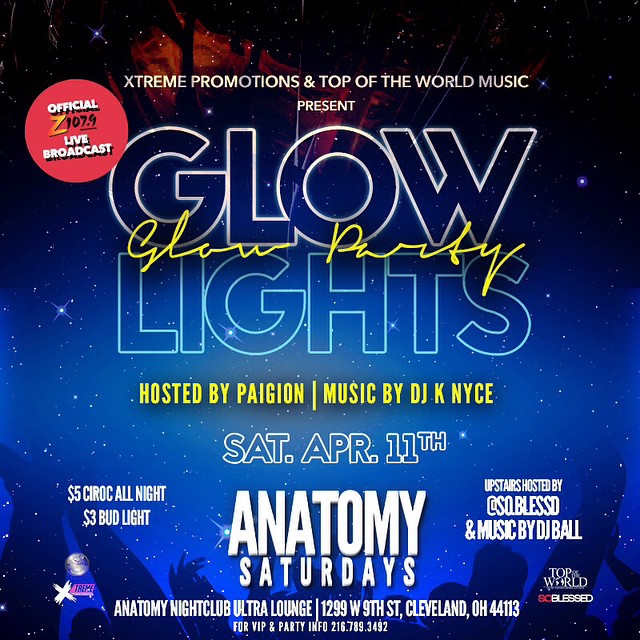This detailed poster for Anatomy Nightclub Ultra Lounge advertises an event called "Glow Lights" presented by Extreme Promotions and Top of the World Music. The vibrant backdrop of the poster features a black-dark blue color palette adorned with numerous white dots, resembling a star-filled night sky. 

At the top left corner, there's a red label marked "Official Z-107.9 Live Broadcast." Adjacent to this, the main title reads "Extreme Promotions and Top of the World Music Present Glow Lights," with the words "Glow Party" elegantly inscribed in yellow cursive between "Glow" and "Lights."

Centered below this title, the event specifics include "Hosted by Pagean" and "Music by DJ K Nice," also notably in yellow. The event is scheduled for Saturday, April 11th, highlighting exciting beverage offers with "$5 Ciroc All Night" and "$3 Bud Light," and is part of the "Anatomy Saturdays" series, suggesting an upstairs party hosted by "@so.dot.blessed" with music by "DJ Ball."

The bottom of the poster provides logistical details, listing the venue's address as "1299 West 9th Street, Cleveland, Ohio 44113," and a contact number for VIP and party info: "216-789-3492." The image also features silhouettes of a dancing crowd at the bottom, enhancing the lively and dynamic atmosphere of the advertised event. 

Additional sponsors, "Extreme" and "Top of the World," are noted on the lower corners of the poster, ensuring a comprehensive promotion for what promises to be an electrifying night at Anatomy Nightclub Ultra Lounge.